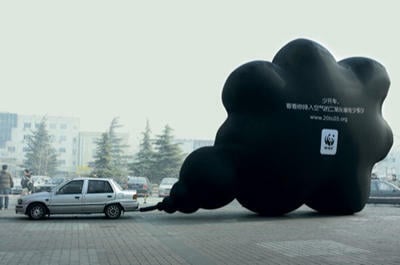A detailed photograph, captured on a foggy day, showcases a light-colored mid-sized car in a parking area. The vehicle is seen in profile, facing left, and is towing an enormous black balloon that resembles a parade float. The balloon, towering approximately five times the height of the car and stretching about four times its length, features a peculiar design with numerous round shapes. Stand-out details include white text in a foreign language and an emblem in the middle that depicts a black and white panda along with the bold letters "WWF" beneath it. Despite the text and an associated URL being blurry and hard to discern, the logos are recognizable. The background includes a row of small-town buildings, additional parked cars, and dark green pine trees, lending a quaint atmosphere to the foggy scene. The foreground consists of paver stones, enhancing the realistic, representational photographic style.